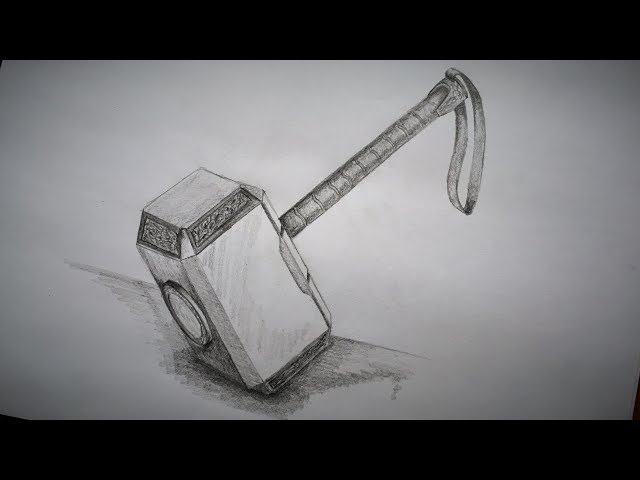This detailed illustration, likely created with pencil or charcoal, depicts a medieval-style mallet reminiscent of Thor's hammer. The mallet rests on an ambiguously outlined surface, perhaps a table edge or the ground, sketched with gentle black and gray lines. The handle of the mallet, adorned with decorative lines, features a looped strap at its end, similar to a strap on a leather-covered steering wheel. The head of the mallet showcases intricate, albeit unclear, decorations that lend a slightly floral aesthetic. The overall rendering gives the impression of a well-crafted art class piece, demonstrating various sides of the hammer with a nuanced shading technique that predominantly covers the paper in shades of gray.